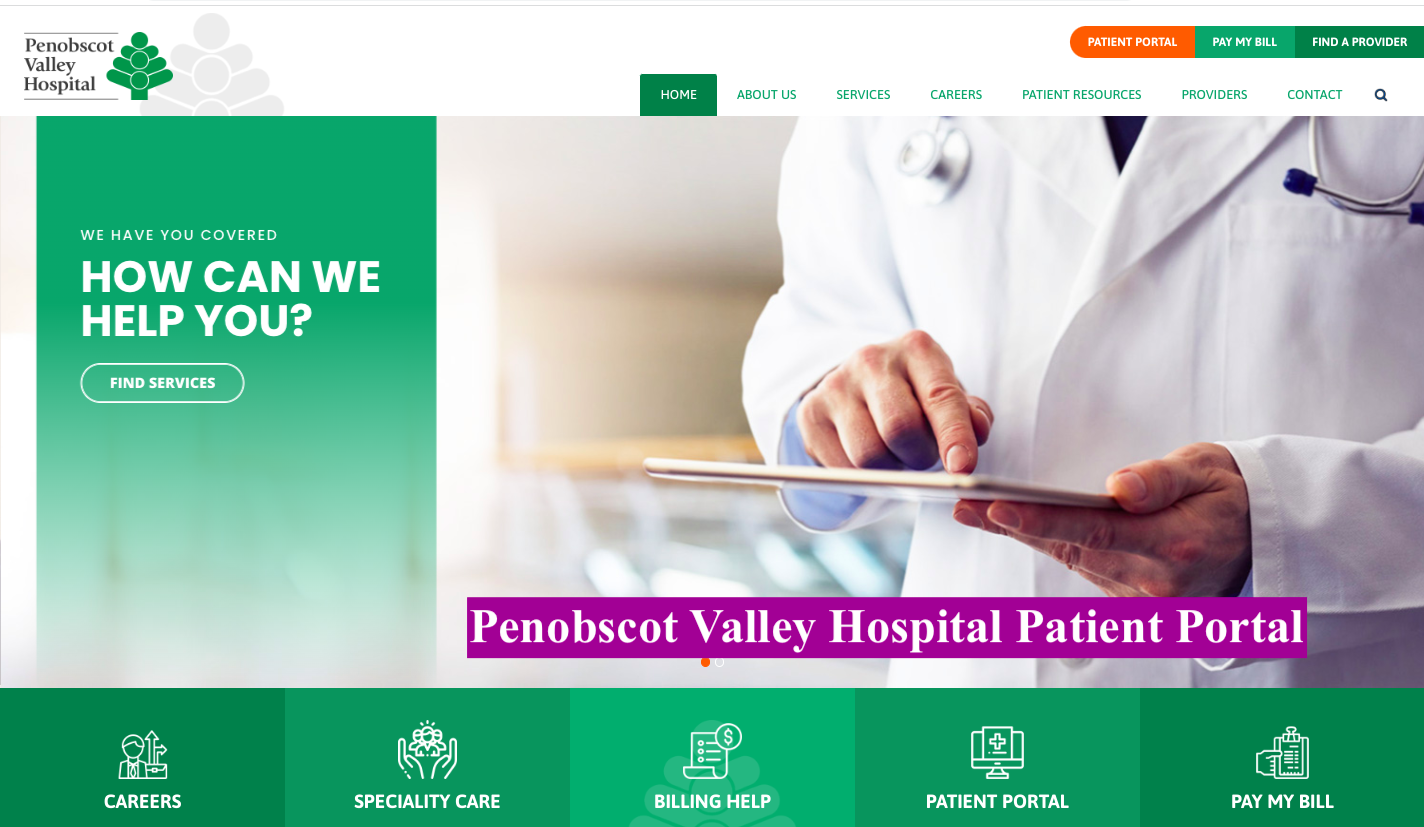This is a detailed screenshot of the Penobscot Valley Hospital homepage, showcasing the hospital’s logo at the top left, which features the text 'Penobscot Valley Hospital' alongside a tree icon. On the top right, there are prominent links in varying colors: 'Patient Portal' in orange, 'Pay My Bill' in dark green, and 'Find a Provider' in dark green as well. Below these links, the navigation bar includes tabs for 'Home,' 'About Us,' 'Services,' 'Careers,' 'Patient Resources,' 'Providers,' and 'Contact,' with a magnifying glass icon for search functionality at the far right.

Dominating the center of the webpage is a large photo of a doctor scrolling on an iPad. Overlaid on the left side of this photo is a green box displaying the text, 'We Have You Covered. How Can We Help You? Find Services.' At the bottom right of the photo, 'Penobscot Valley Hospital Patient Portal' is highlighted in white font against a purple background.

Towards the bottom of the page are icons representing key areas of interest, each labeled as 'Careers,' 'Specialty Care,' 'Billing Help,' 'Patient Portal,' and 'Pay My Bill,' providing quick access to essential hospital services.